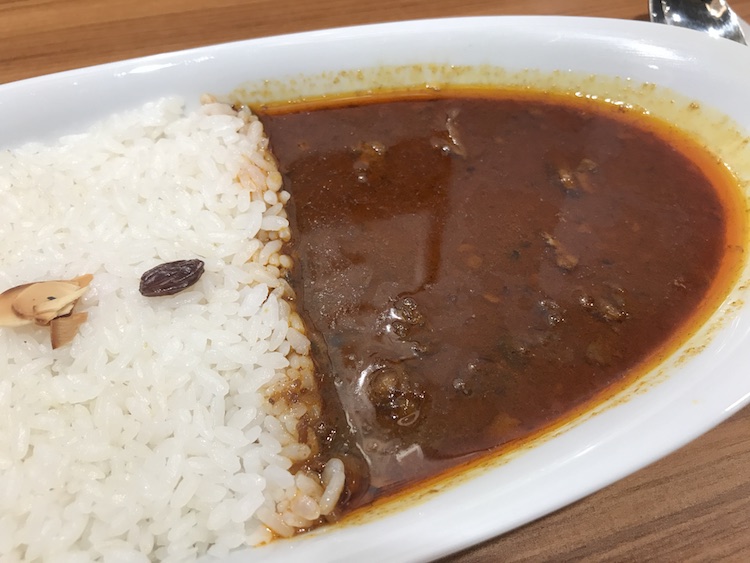A partially visible white plate, set on a medium brown wooden table with varied shades, holds two distinctly separate types of food. On the left side of the plate, there is a precise edge of white rice, garnished with a raisin and a possible slice of mushroom. To the right, a dark, runny beef curry with floating chunks occupies the space, resembling a thin gravy. The wood grain of the table appears almost black in some areas and runs horizontally. In the top right corner of the image, a silver spoon is partially visible.